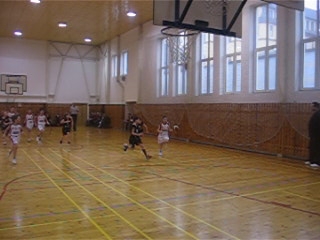In this image, an indoor gymnasium, likely part of a high school, serves as the backdrop for a lively basketball game between two teams of children. The gym's roof features round, circular lights built into it, casting a bright glow on the playing area below. One of the walls is lined with mirrors, which are covered by a protective netting. 

On the court, two basketball hoops are visible, indicating an ongoing competitive match. The children are divided into two teams, distinguished by their jerseys—one team dons white, while the other wears black. The gymnasium's floor, made of brown springform material, is marked with yellow and red lines that outline the basketball court's boundaries and key areas. Despite the small size of the image, the energetic atmosphere of the game is palpable, even though the basketball itself is not visible in the frame.